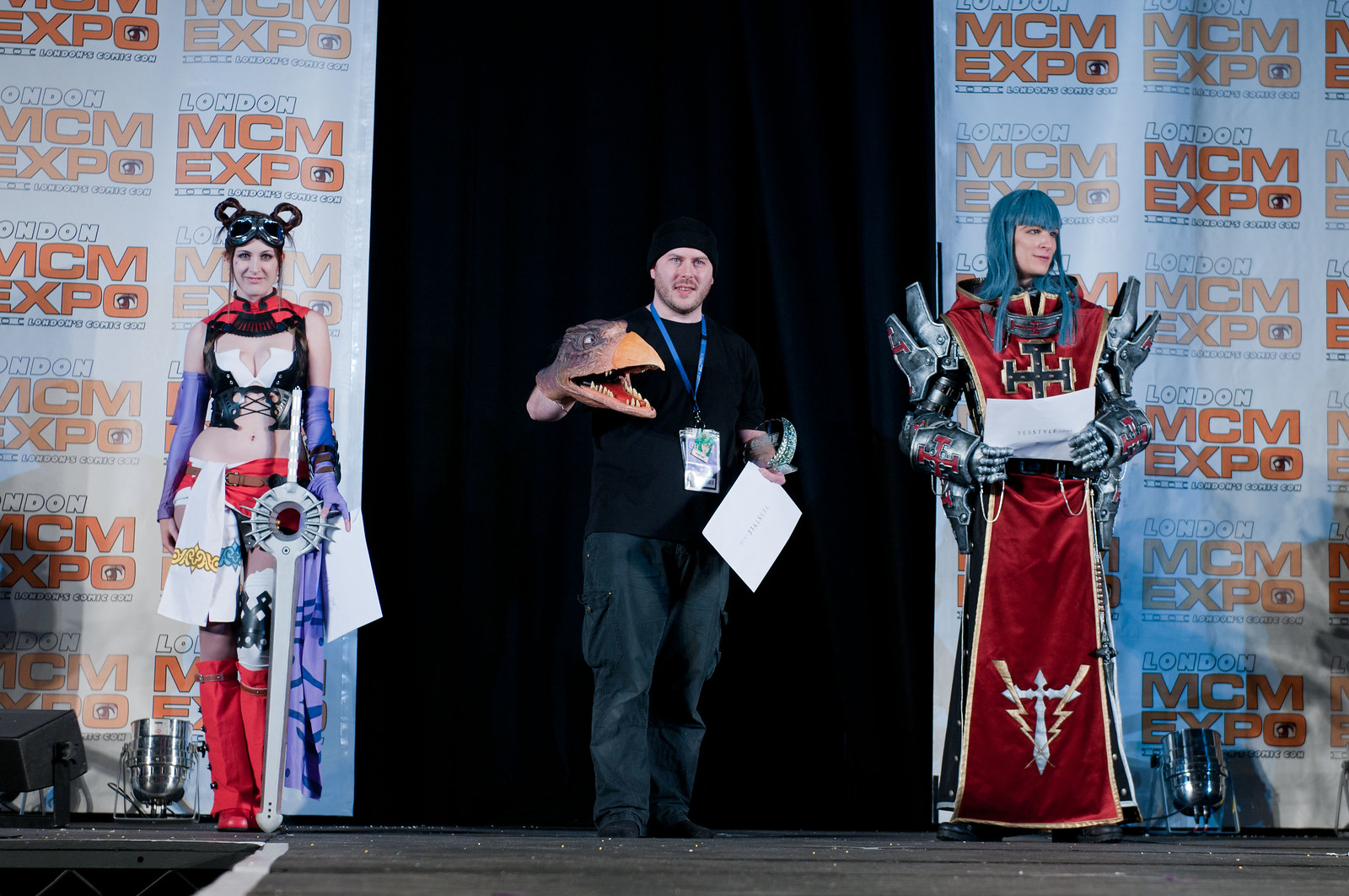This detailed image captures a stage scene from the London MCM Expo, often referred to as London's Comic Con, featuring a cosplay presentation. The horizontal composition showcases three individuals in elaborate costumes. On the left stands a female cosplayer adorned in a futuristic knight outfit, complete with red boots, a black and white midriff-baring top, purple sleeve, goggles perched atop her head, and her hair styled into two buns. She brandishes a sword with a sleek, advanced design. To the right, another female cosplayer flaunts a long, red, sci-fi inspired dress with blue hair and armored arm pieces, exuding a commanding presence. Positioned in the center is a male figure, differentiated by his casual attire consisting of a black shirt and blue jeans. He intriguingly wears a dark hat and a prominent badge hanging down his neck while holding a white piece of paper in one hand. His other hand features a distinctive puppet resembling a dinosaur or bird head, adding a curious element to the scene. They are set against a varied backdrop, with the two cosplayers framed by separate panels, and the man in the middle against a dark background, suggesting a focal point on his peculiar prop during their act.